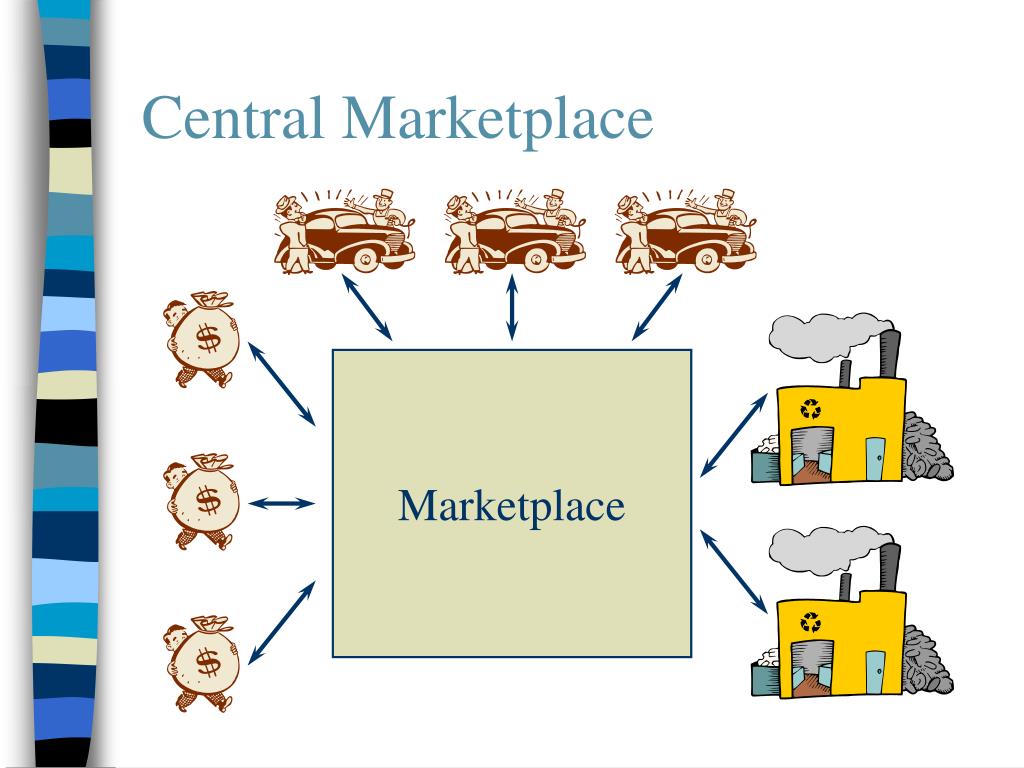This image appears to be a PowerPoint presentation slide featuring a central theme titled "Central Marketplace." The background is white, with a colorful strip of stripes in varying shades of black, blue, beige, and white on the left-hand side. Prominently displayed in the center is a beige square with blue text that reads "Marketplace." Above this square, "Central Marketplace" is also written in blue text.

Surrounding the central "Marketplace" square, arrows point to and from various cartoon illustrations that depict different scenes. On the left side, there are three illustrations of men holding large sacks with dollar signs on them, symbolizing transactions or money exchanges. Across the top, there are three scenes featuring an old-fashioned car with people standing around it, likely indicating car sales or negotiations. On the right side, there are two illustrations of yellow factories with gray smokestacks and piles of recyclable materials, such as paper and tires, illustrating recycling facilities.

Together, these elements suggest a life cycle or flow of activities that revolve around the central marketplace concept, possibly focusing on commerce and recycling.